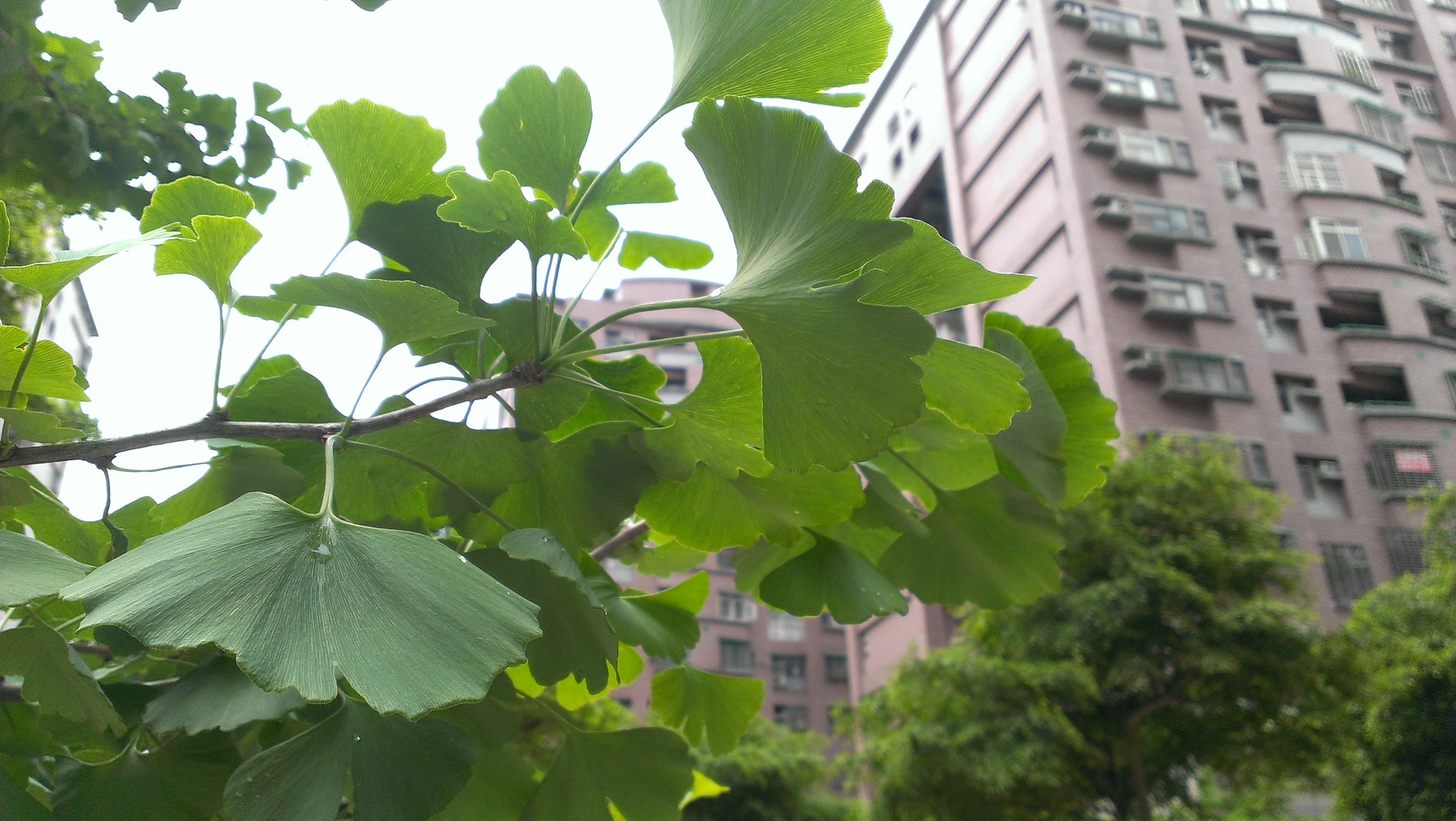This image captures a scene with a distant view of a tall, mauve-colored apartment or hotel building, which appears to be at least 10 stories high. The building, featuring numerous two-pane windows and balconies concentrated on one corner, stands against a white, overcast sky. In the foreground, lush green foliage dominates the view, including a vine, ferns, and a variety of other plant types. Two additional trees are also partially visible but appear blurrier and are set further back. Two distinct buildings can be discerned behind the dense foliage, adding depth to the scene. The overall composition is horizontally oriented, with a close-up of the vine and broad leaves prominently in the front, framing the urban landscape in the background.